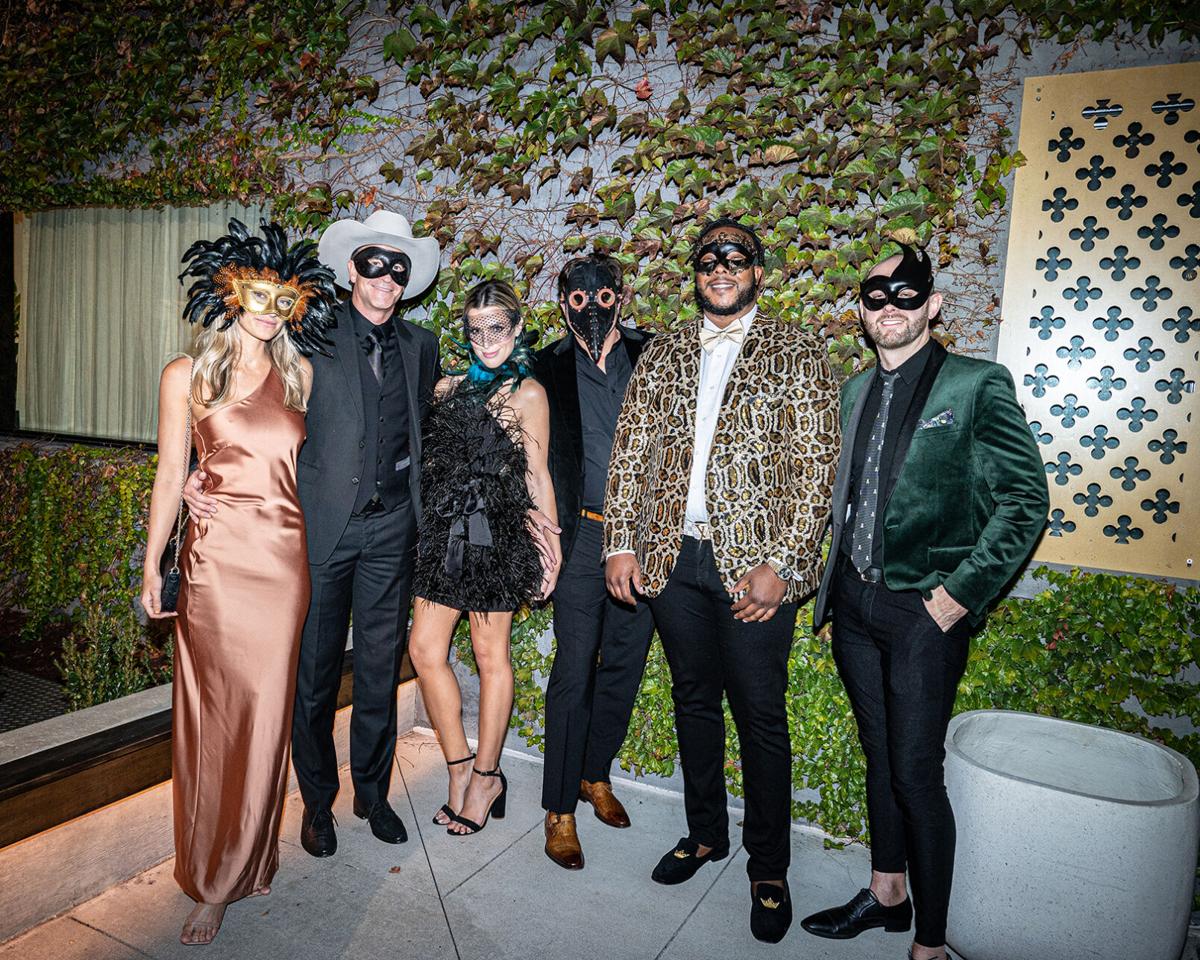This candid photo captures six friends at a masquerade party, posing in a garden in front of an ivy-covered building. On the left, a blonde woman in a copper-colored dress with a gold mask adorned with black and brown feathers stands barefoot. Next to her, a man dressed in all black except for a white cowboy hat and a black Lone Ranger-style mask poses confidently. Beside him, a woman clad in a short feathered black dress and high heels wears a delicate net mask and holds the hand of the man next to her. This man is costumed in a black suit with a plague doctor mask, accessorized with a brown belt and shoes. To his right, a man sports a loud leopard-print jacket, black pants, and a small matching face mask. On the far right, a man in a green velvet jacket and black pants with no socks, completes the group with a black wispy mask. The background features windows with curtains and a patterned design reminiscent of playing card spades, further setting the scene for this glamorous and mysterious event.